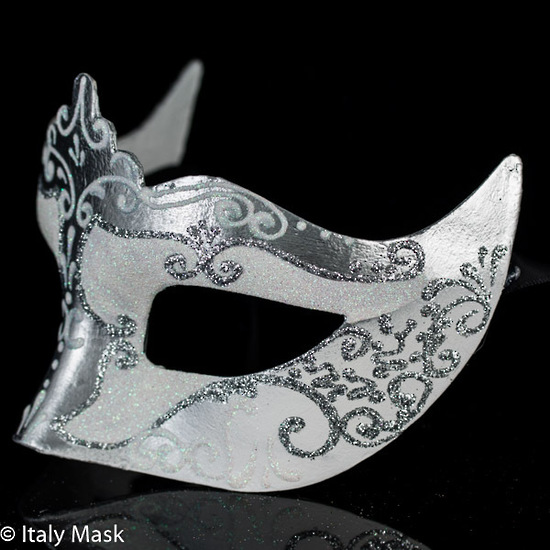This close-up photograph captures an elegant masquerade-style eye mask in exquisite detail. The mask, predominantly a light silvery gray that nearly appears white, features intricate, darker silver curvy etchings that add a delicate, ornate touch. The design includes a shinier silver nose bridge and accents around the eye openings, enhancing the mask's luxurious appearance. It sits on a reflective black surface, likely glass, which mirrors the mask below and creates a seamless blend into the pitch-black background. In the bottom left corner, white text reading "Italy mask" is prominently displayed, indicating either a trademark or the mask's origin. The overall composition underscores the mask's sophistication and the craftsmanship of its intricate embellishments.